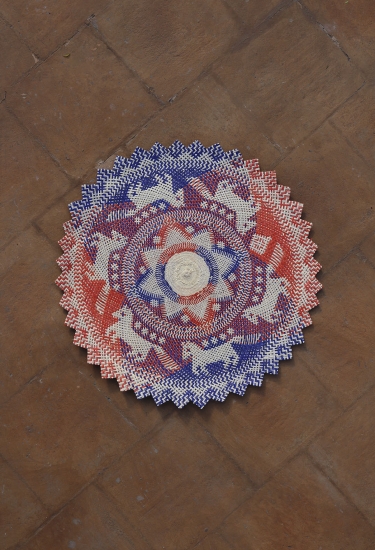This image depicts a meticulously detailed round rug set on a terracotta tile floor. Its design emulates traditional indigenous patterns, though not handcrafted by indigenous artisans. The rug's striking palette includes deep blues, muted and vibrant oranges, reds, purples, and creams, which blend together in a captivating gradient. The outer edge of the rug features a jagged, triangular border reminiscent of saw teeth.

Encircling the rug's center is an intricate pattern of six white horses, each adorned with four small stars running along their backs, creating a sense of dynamic motion as they trot in unison. These horses are set against a rich backdrop of gradient hues.

At the heart of the rug lies an exquisite design that could be interpreted as a flower or a radiant sun, marked by symmetrical golden petals surrounded by diamond shapes. This central motif is enclosed by a gold circle, enhancing its brilliance. The rug's overall design is a harmonious blend of indigenous-inspired artistry and vibrant, contrasting colors, making it a standout piece in its rustic setting.